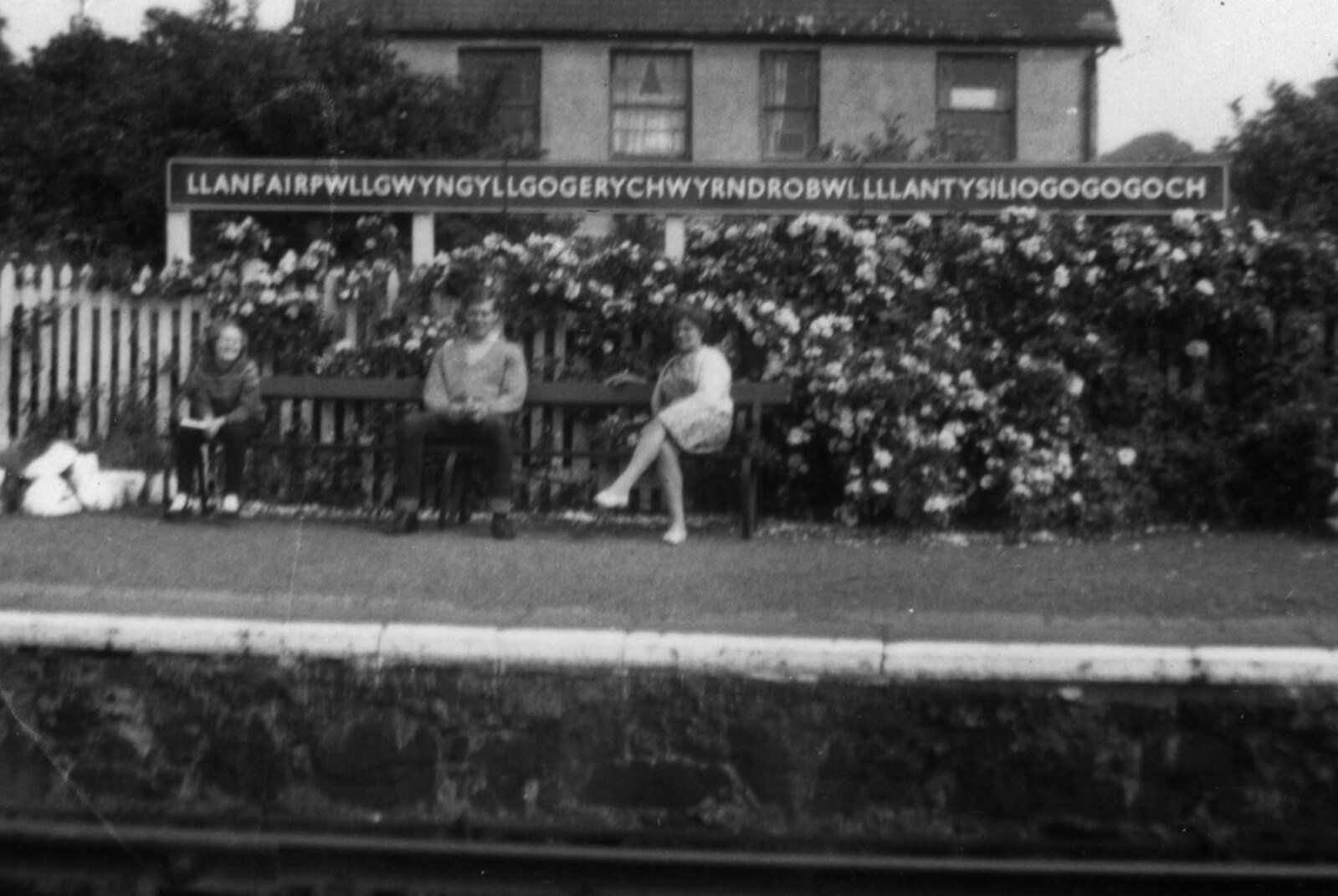This black-and-white photograph captures a nostalgic scene at what appears to be a train station. In the foreground, along the bottom edge, there's a partial view of a stone wall with a flat, paved area in front of it. Seated on a large wooden bench above the wall are three individuals. On the left, there's a younger person, possibly a woman, with something between their legs that resembles handlebars, suggesting a tricycle or similar small wheeled apparatus. Next to them, in the middle, an older man is wearing a sweater. To the right, a woman dressed in a dress sits cross-legged. Behind the bench, a white picket fence laden with blooming flowers runs the length of the scene. Further back, an old brick building is visible through the floral barriers, adding to the charm of the setting. A prominent sign hanging above the fence displays an incredibly long name: "LLANFAIRPWLLGWYNGYLLGOGERYCHWYRNDROBWLLLLANTYSILIOGOGOGOCH," making a striking impression with its complexity and length. Although the photograph is out of focus, the interaction between the subjects and the historical ambiance of the location come through vividly.